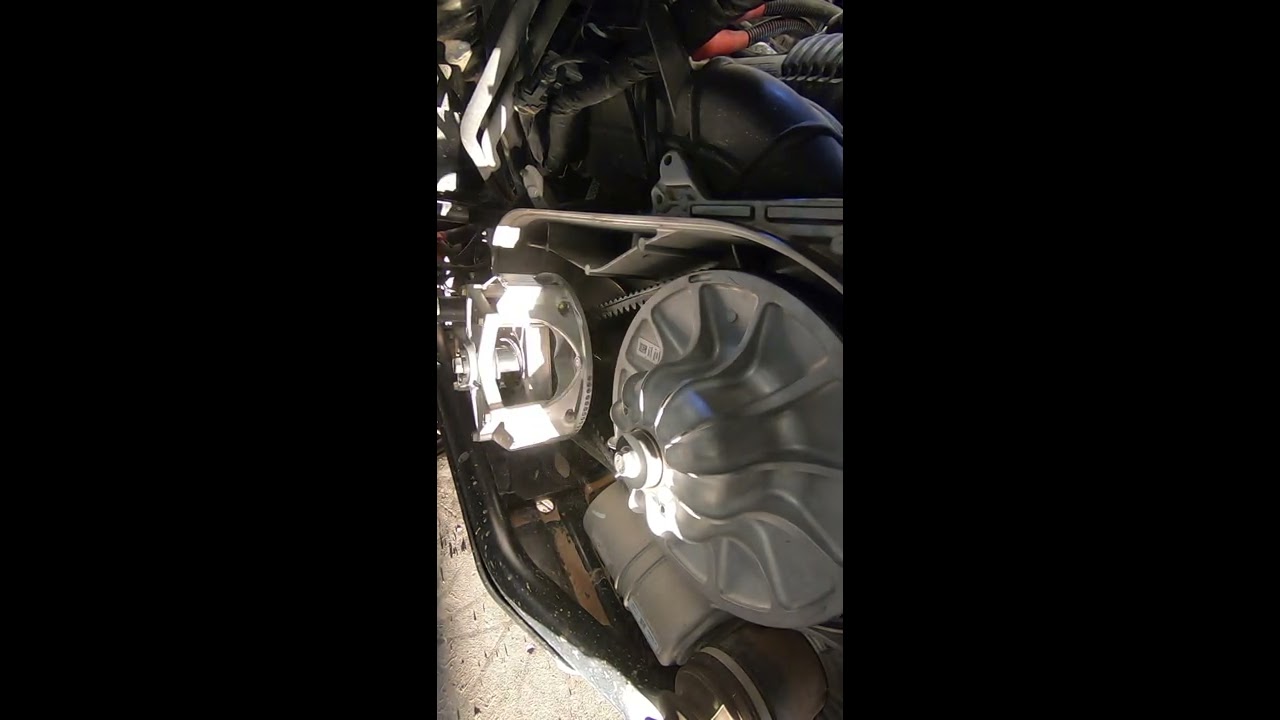The image features a close-up view under the hood of a car, focusing primarily on the engine components. The middle section of the image prominently displays a large silver or chrome cylindrical device, potentially an engine part or mechanical segment. Adjacent to it is a smaller silver round piece with symmetrical segmentation, possibly connected by a bolt or screw. Several black tubes are visible, intricately weaving through the metallic parts, with a particularly large tube running from the center to the center-right. The image also captures faint red elements near the top and some obscure metal structures, indicative of complex machinery. Beneath these elements, a black object with a white stripe or another machinery part can be partially seen. The image is tightly cropped vertically with dark black borders on both the left and right sides, suggesting it was likely taken with a smartphone.